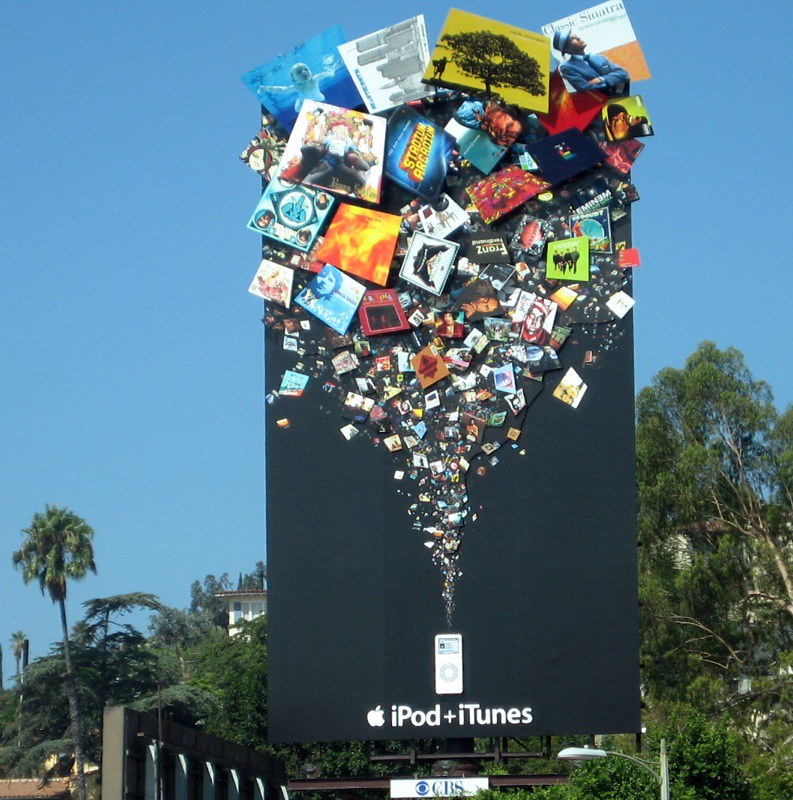The billboard features an elongated rectangular sign primarily colored in black. At the bottom center of the sign, the text "iPod + iTunes" is displayed in white font, accompanied by the Apple logo to its left. Above this text, an iPod is depicted, positioned as if it is releasing a vibrant spray of images. These images, starting small and growing larger as they move upward, include the fronts of CD labels, record labels, and various album covers, suggesting a dynamic burst of musical diversity. The overall design visually represents the extensive music library available through iPod and iTunes, using the spray of images to convey the diversity and volume of content available.